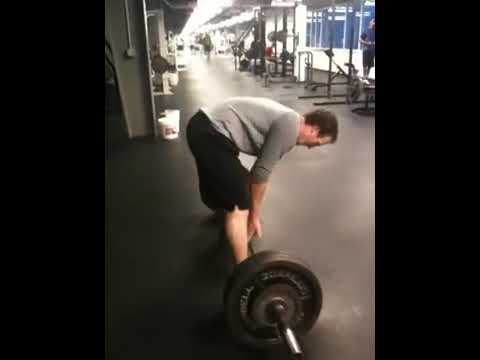In the photograph, a man is indoor lifting a heavy weight within a spacious, well-equipped gym. Positioned centrally, he is bent at a 45-degree angle at the waist, preparing to lift a large black dumbbell with a silver bar, which features white, but illegible, writing on its visible end. His appearance includes short dark brown hair and a clean-shaven face. He is dressed in black shorts and a gray long-sleeve shirt with rolled-up sleeves stopping at his elbows. The gym itself extends deeply into the background, populated with various exercise machines, likely treadmills and weight benches, gradually diminishing in size with the perspective. The lighting sources appear to be on the right side of the frame, illuminating part of the scene while leaving the left side in shadow. In the distant background, there's a faint image of another individual, though details are indistinct. The floor of the gym is a grayish color, and there are black rectangular framings on the left and right sides of the image.